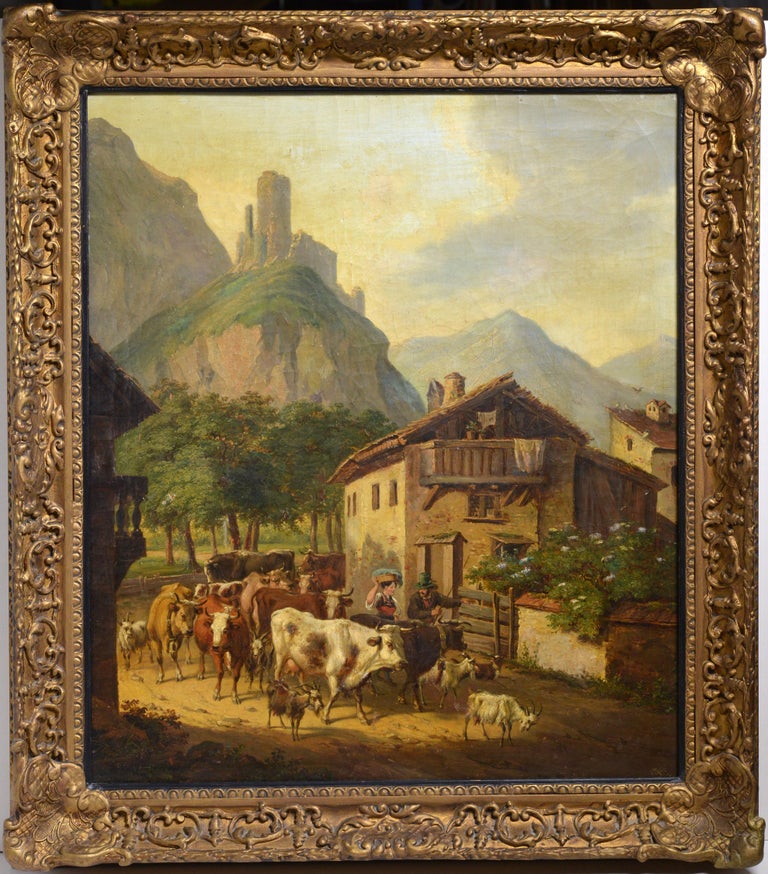The image depicts a detailed and picturesque painting of a rural village scene, encased in an ornate, gilded gold frame characterized by intricate carvings featuring flowers, leaves, hearts, and scrolling designs. The painting, which has a realistic style and appears to be quite old—suggestive of the 1800s or 1900s—is set within a vertical rectangular format, bordered by thin black strips on the top and bottom, and thin gray strips on the sides. 

In the center of the scene, a herd of around 10 to 15 cattle, including brown, black, yellow, and brown-and-white cows, and a few baby calves, meander down a village street. Two villagers, possibly a man and a lady carrying something on her head, guide and feed the animals. There are also some goats accompanying the herd. The village itself features two-story houses, with the most prominent house displaying a balcony on the top floor and thatched or wooden stick roofs with adobe brick walls.

Surrounding the village are lush green trees and mountainous terrain with light brown hues. The sky above is lightly colored with shades of blue, gray, and yellow, adding to the overall pastoral and tranquil atmosphere of the painting.